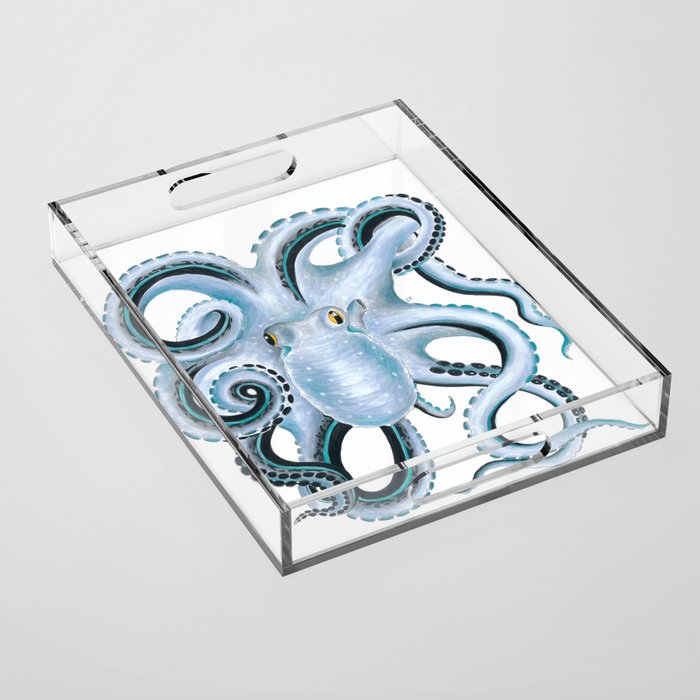This detailed color photograph showcases an acrylic serving tray set against a light gray background. The tray, viewed from above, features a flat bottom with a lip about two inches high, culminating in clear handles on either side. The bottom of the tray is adorned with an illustration of a large, pale blue octopus, outlined in black and accented with shades of green and navy blue. The octopus, which occupies the entirety of the tray's base, has prominent yellow eyes and detailed black suckers on its tentacles that extend to the left and right edges. The character of the octopus appears approachable and friendly, enhanced by small white dots on its face. The acrylic material of the tray creates a subtle prism effect, adding dimension to the scene, as the handles seamlessly blend into the tray’s transparent sides. This meticulously arranged photograph makes the tray appear as though it's featured in a high-end magazine.